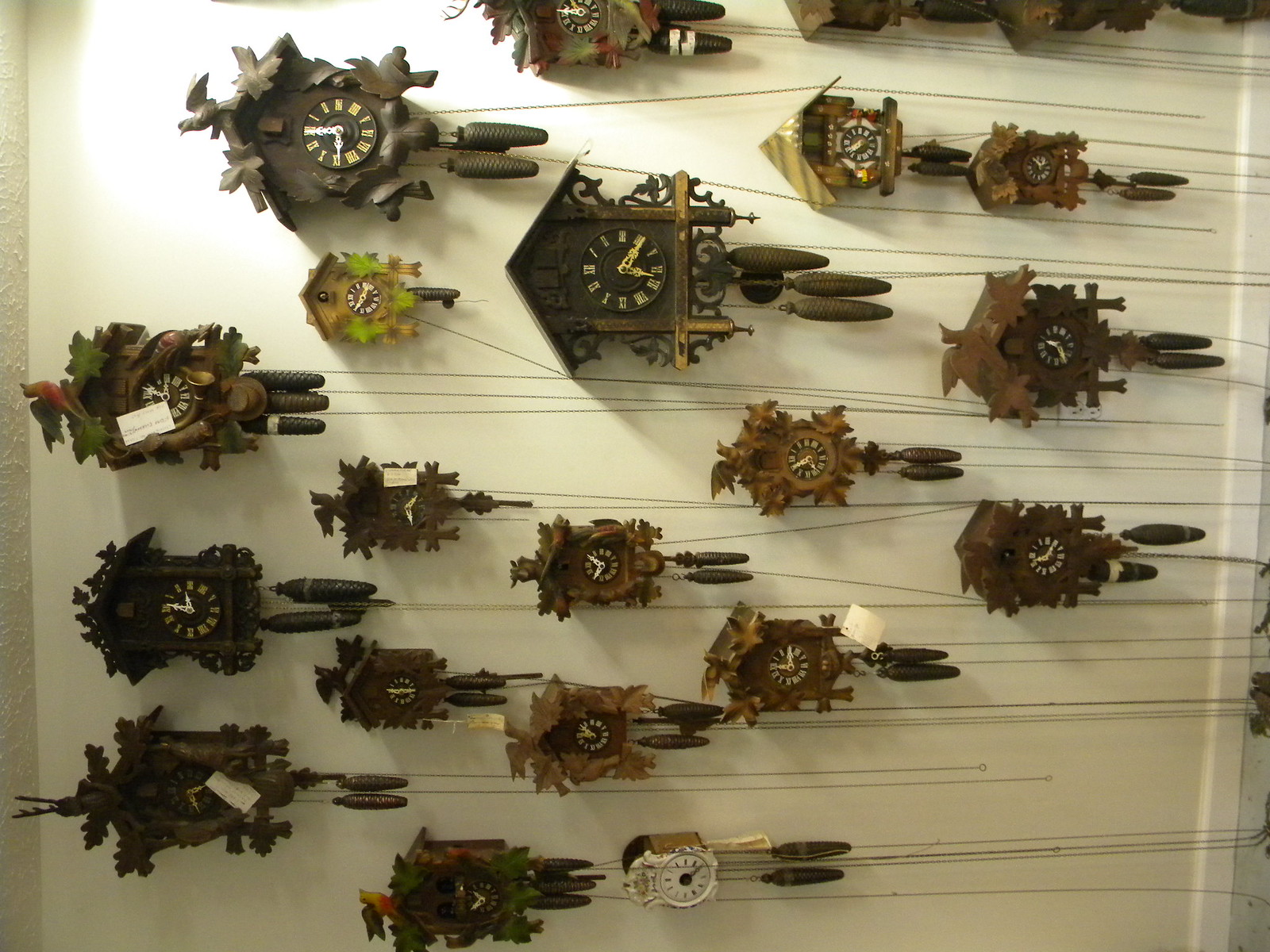The image depicts a collection of approximately 15 cuckoo clocks of various sizes and designs, all mounted horizontally on an off-white, stucco-like wall. The clocks are primarily in shades of brown, from dark to light, with some featuring green accents or carved cuckoo birds on top. One clock stands out with its white and green coloration. The clocks' hands point to different times, and from each hangs dark, pinecone-like weights attached to chains, which dangle toward the right side of the image. Some clocks have white price tags indicative of retail sale. Shadows cast by the chains add depth to the scene, and a cream-colored molding is visible along the right edge of the photograph. Note that the photograph is rotated 90 degrees counterclockwise, making the clocks appear sideways.